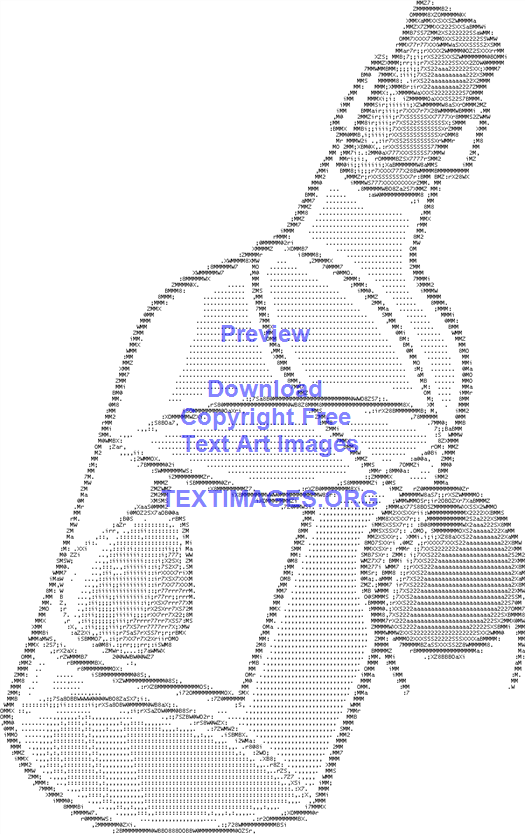The image features a pixelated depiction of a wine bottle on a grayscale background, composed entirely of various keyboard characters, such as letters, numbers, and symbols including A's, 2's, M's, and asterisks. The bottle, which is angled slightly to the right and capped with a cork, has a label featuring a prominently displayed pear. Additionally, there appears to be a ball hanging off the bottle, attached by a rope. The whole image has a cartoony and somewhat disproportionate style. Overlaid in light blue text across the middle of the bottle are the words "Preview, download copyright-free text art images," followed by "textimages.org" at the bottom.